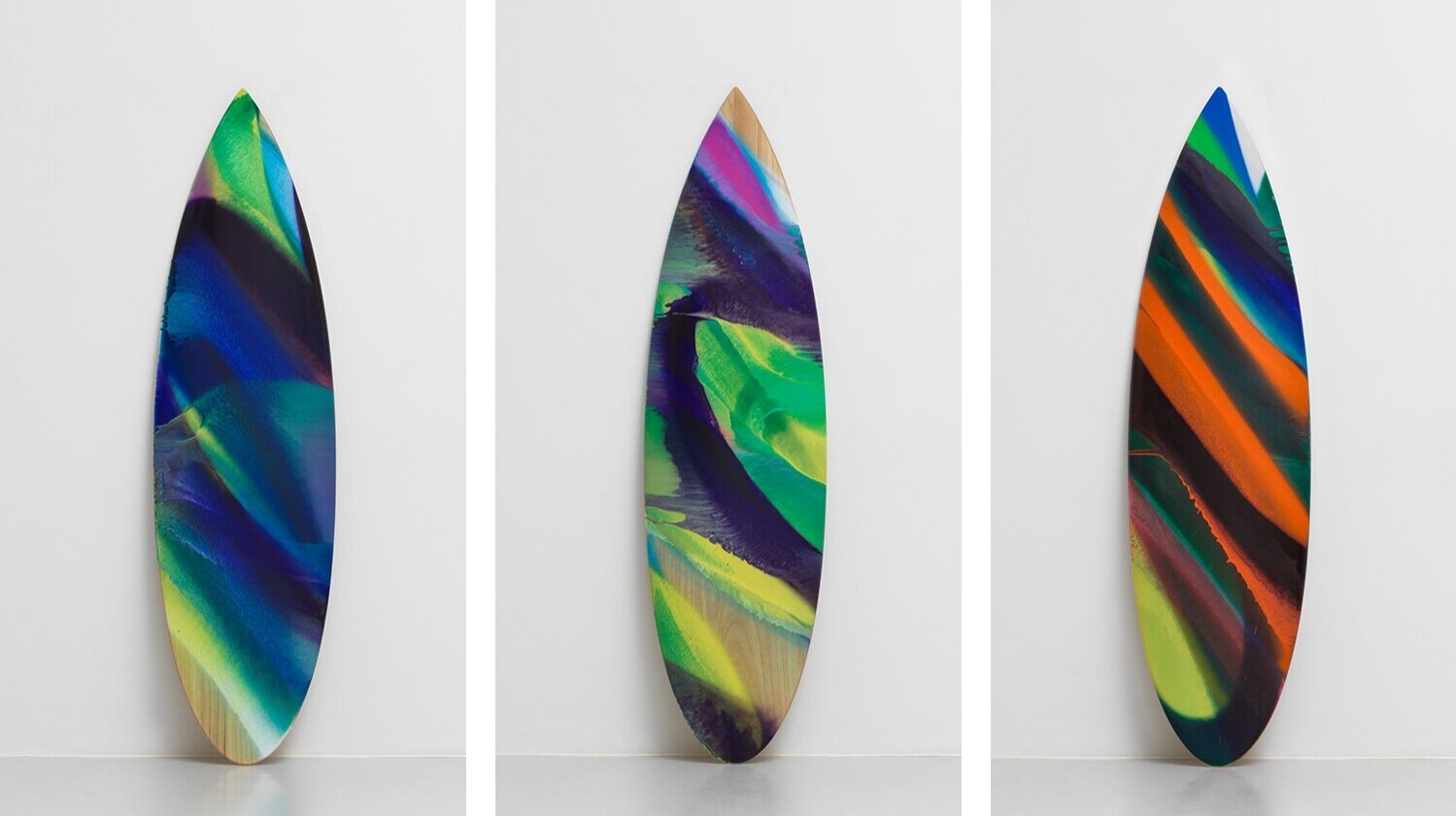The image showcases three distinct surfboards standing upright, each in a separate rectangular panel against a solid white floor or countertop. Each surfboard has a unique, multicolored design but shares a white background that highlights their vibrant patterns. 

On the left, the surfboard features a primarily green and blue swirl with accents of yellow and brown, revealing some of the natural wood texture. In the middle, the surfboard exhibits a blend of black, purple, green, and yellow swirls with visible wood patches at both the top and bottom. The surfboard on the right is the most striking with bold and colorful stripes, predominantly featuring orange, but also includes blue, green, black, yellow, red, and light blue.

All three surfboards are of the same size and shortboard shape, meticulously designed to stand out with their vivid, swirling colors and contrasting stripes, creating a visually captivating trio displayed in equally sized, tall rectangular images. No text is present in the image.